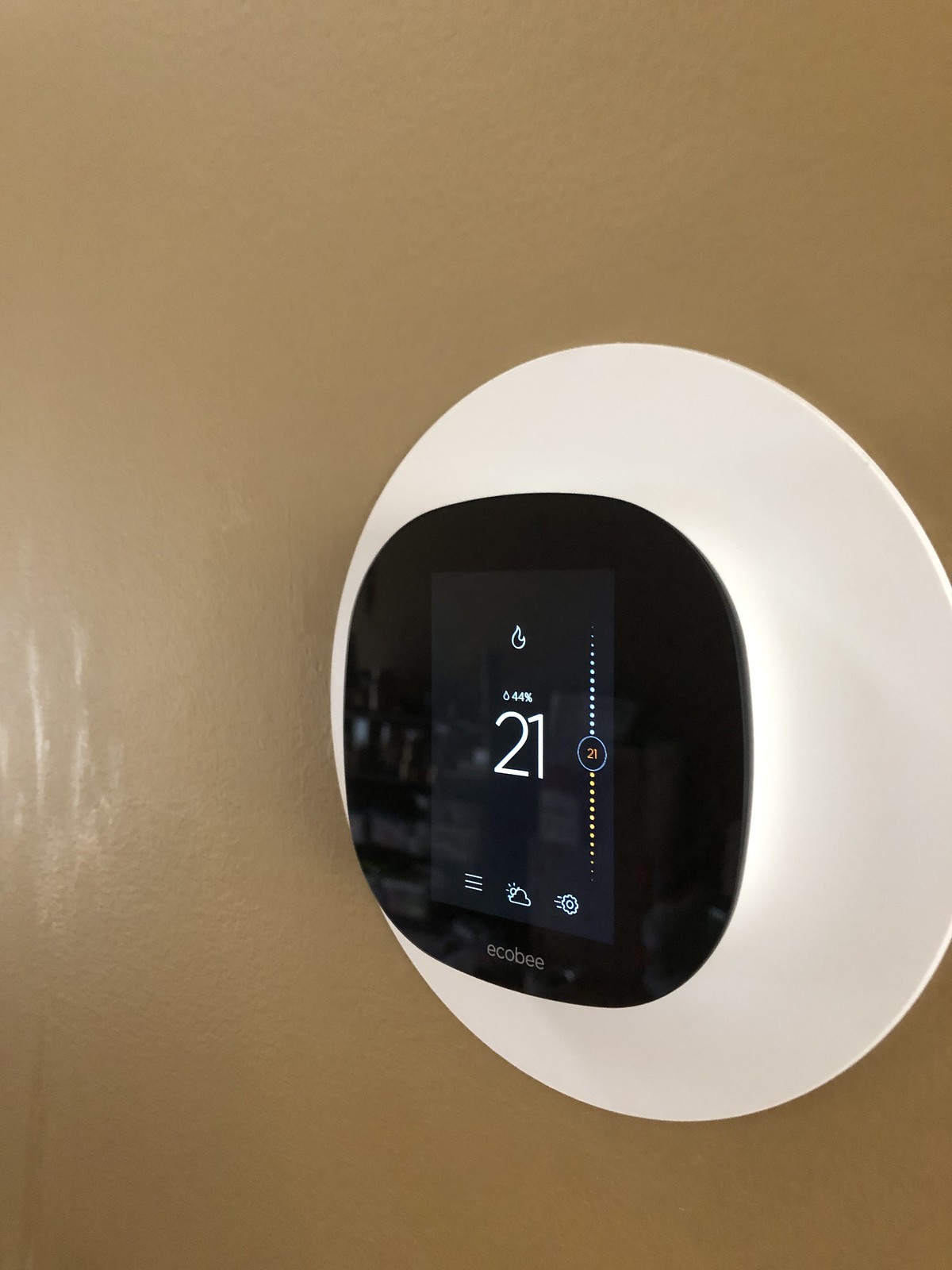The photograph features a sleek, modern, upscale digital thermostat mounted on a medium brown wall with a flat paint finish. On the left side of the image, there are streaks that suggest someone touched the wall while the paint was still wet, leaving a subtle handprint. The thermostat, located on the right side of the image, is a white, round plastic device with a black LED screen that has a rounded-edged square shape. At the bottom of the screen, the brand name "ecobee" is prominently displayed in white print.

The screen itself displays several icons and readings. At the top, a small fire emblem is shown twice, followed by the text "44%" and "21" beneath it, both in white. To the right of these numbers, there's a dotted line, with the top dots in white and the bottom dots in yellow. An orange circle next to these represents the number "21." 

Below these main displays, there are three option icons: three horizontal lines indicating an additional menu, a gear symbol for settings, and a cloud with the sun peeking over it, likely representing weather information or brightness settings.